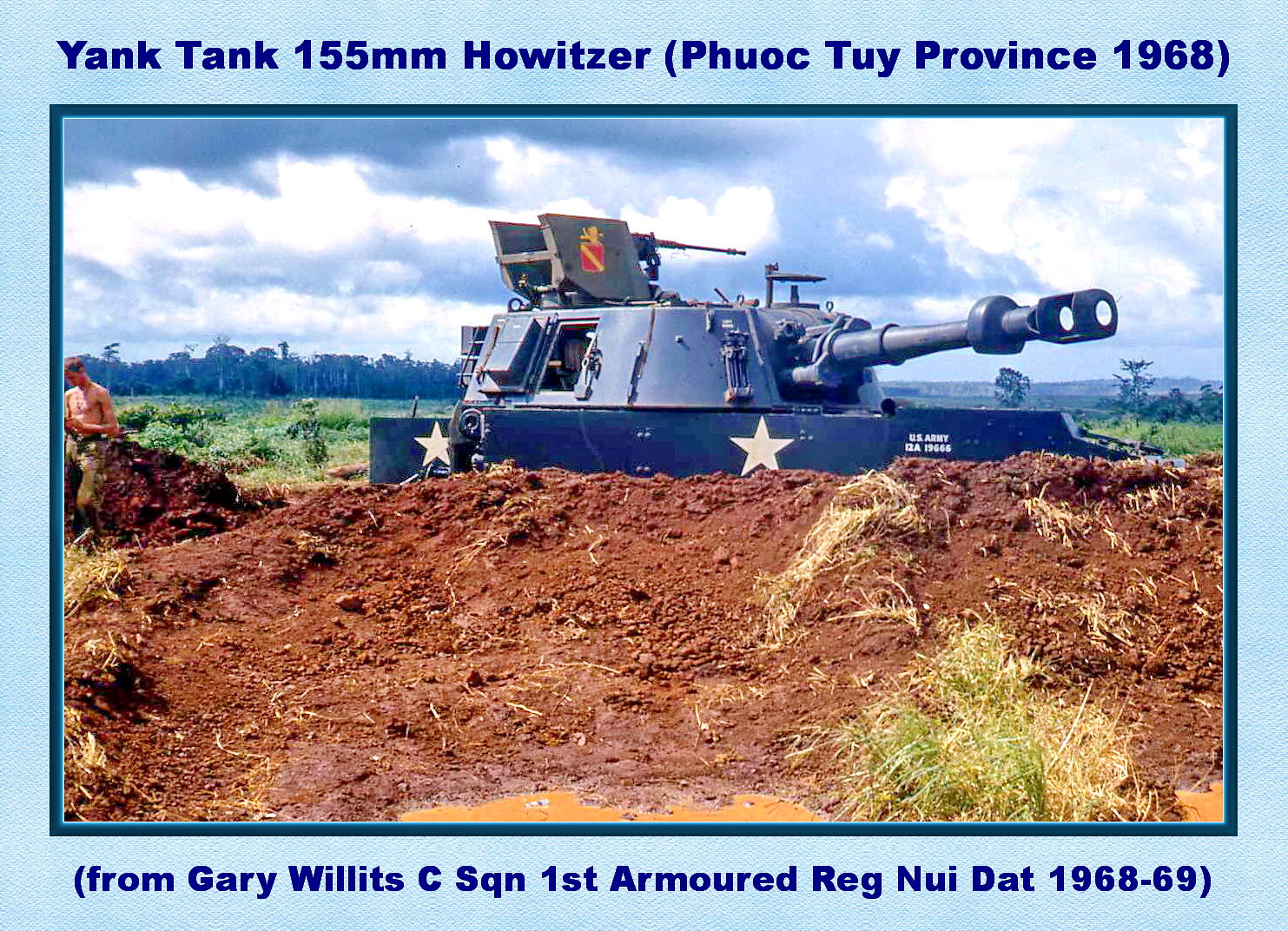The image is a color photograph from the Vietnam War era, showcasing a large tank, specifically a 155mm Howitzer, partially obscured behind a hill of dirt, creating a sense of camouflage. The tank is situated in a grassy area, with trees and a sky dotted with white clouds in the background. The photograph has text overlay at the top, reading "Yank Tank, 155mm Howitzer, Phuoc Thuy Province, 1968," and at the bottom, it says "From Gary Willits, C.S.Q.N. 1st Armored Reg, Nui Dat, 1968-1969." The text is mostly in blue. Additionally, a small body of water is visible at the bottom of the image. This information suggests the photo was taken in Vietnam during the specified time period.